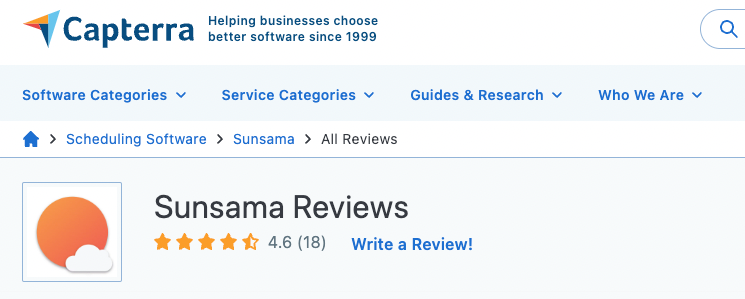In the upper-left corner of the image, there is a graphical element resembling a slightly diagonal blue and pink triangle, with a darker blue hue accentuating its design. Adjacent to this, the word "CAPTERRA" is prominently displayed in bold, black text. Directly to the right of this text, a tagline reads, "Helping businesses choose better software since 1999."

Below this section, there are several navigational categories listed in blue text: "Software Categories," "Service Categories," "Guides and Research," and "Who We Are." 

Further down, the image features a small graphic of a blue house, accompanied by a right-pointing arrow and the label "Scheduling Software." Another right-pointing arrow follows, leading to the name "SunSama." The words "All Reviews," highlighted in black text, are underscored by a thick horizontal line.

To the left of this line, there is a square image containing a pink circle with a white cloud positioned in the bottom-right corner. To the right of this image, bold black text reads, "SunSama Reviews," accompanied by an illustrative rating of four and a half out of five stars, rendered in orange. Adjacent to the stars, there is a numeric rating of "4.6," followed by the number of reviews in parentheses "(18)." A prompt to "Write a Review!" is highlighted in blue.